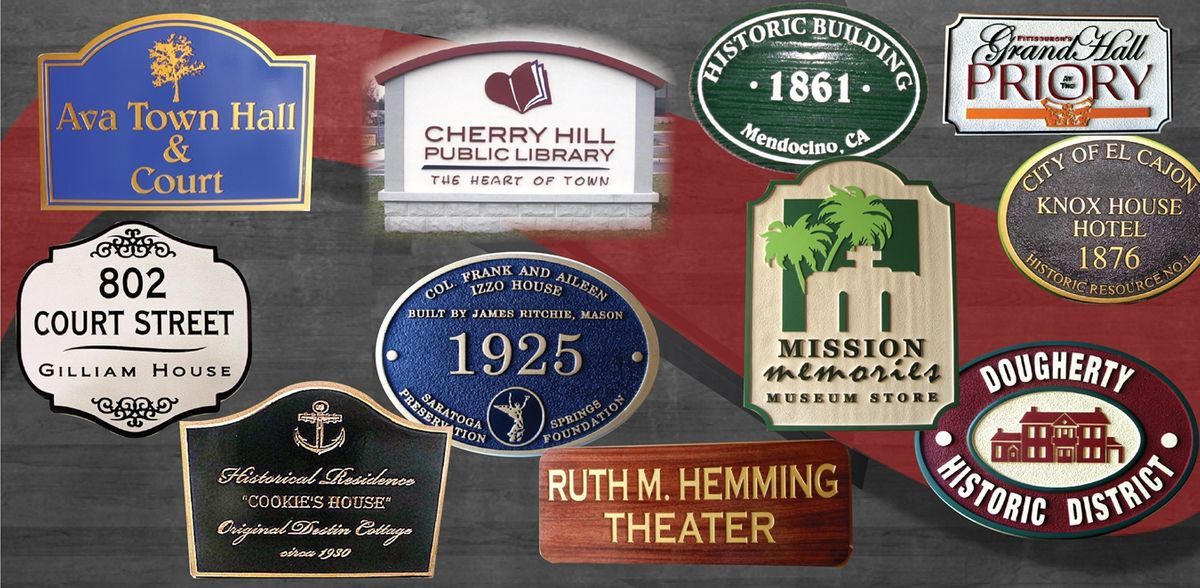The image is a meticulously crafted collage of various signs, plaques, and medallions, each depicting historic and notable buildings, arranged against a gray background accented with a striking red stripe. In the upper left corner, the signs read "Ava Town Hall and Court," "Cherry Hill Public Library," and "Historic Building, 1861, Mendocino, California." Centrally featured, the collage includes "Grand Hall," "802 Court Street," "Gilliam House," "Doherty Historic District," "1925, Colonel Frank and Eileen Izzo House," and "Mission Memories." At the bottom, noteworthy signs include the "Ruth M. Hemming Theater" and the historically significant "Cookies House." The diverse signs, varying in color, material, and style, contribute to the artistic presentation of historically important locations, encapsulated in a visually cohesive and informative arrangement.